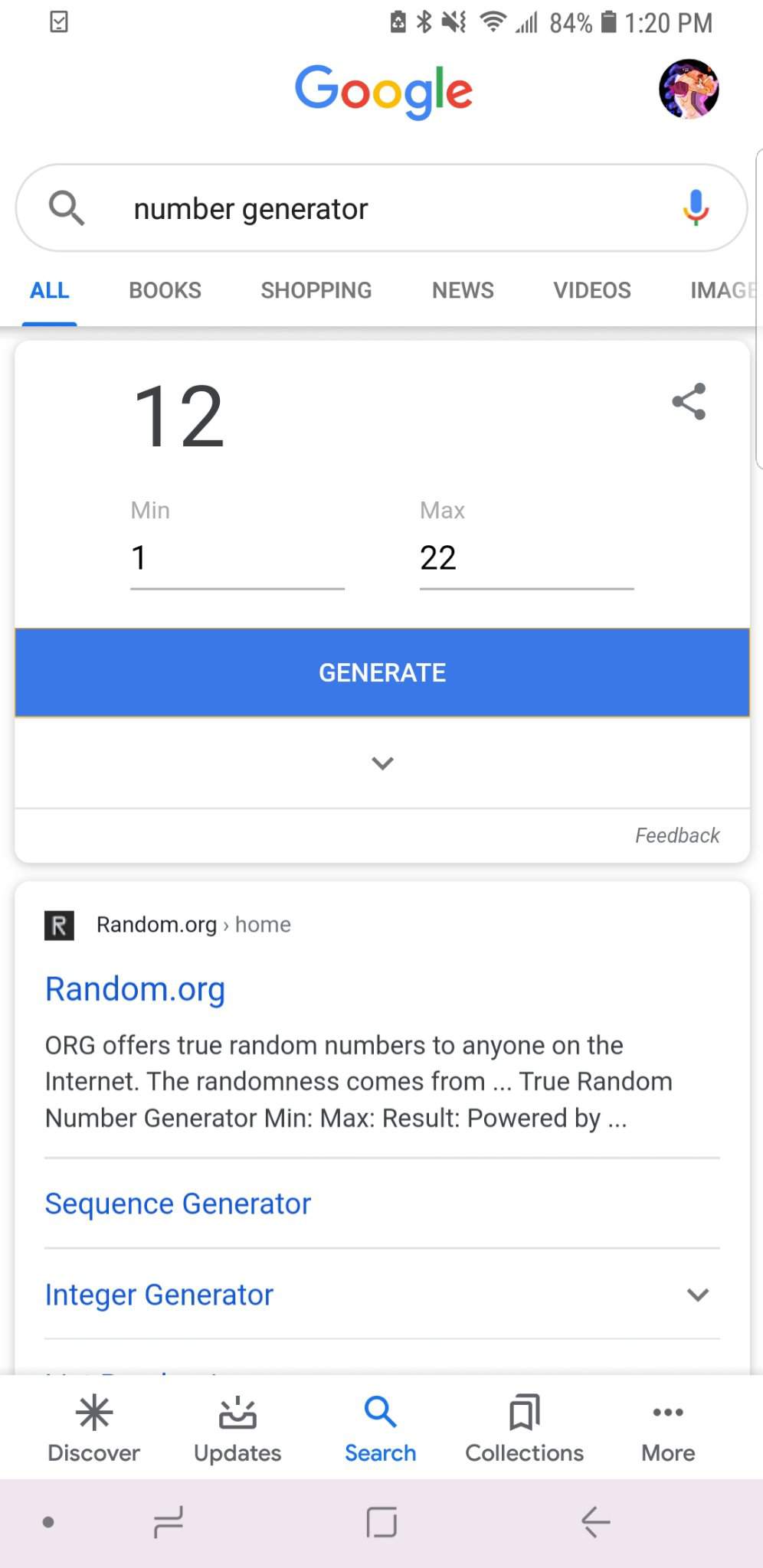The image depicts a Google search results page with the query "number generator" entered in the search bar. Prominently displayed in the results area is Google's built-in number generator tool. The current settings of the tool have a minimum value of 1 and a maximum value of 22, with the generated number being 12. Below the number generator, the first search result appears from random.org, a well-known random number generation website. This result offers additional tools such as a sequence generator and an integer generator, providing users with various options for generating random numbers.